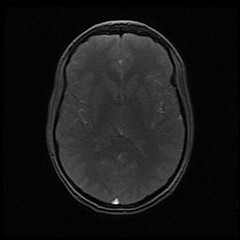The image appears to be an X-ray or a CT/MRI scan of a human brain viewed from above. It features a square-shaped black background with a grayish, semi-transparent representation of the exterior skull in the center, resembling either a skull or an egg. Inside the skull, the scan reveals intricate, fine details of the brain's structure, showing the two hemispheres with various shades of black and gray, indicating different brain tissues or regions. Vein-like or neuron-like patterns are visible, suggesting the complex network within the brain. Notably, there is one pronounced white speck at the front and several smaller white specks scattered throughout the image, which might indicate points of interest or potential injury. The overall appearance is abstract, emphasizing the detailed and textured nature of the brain's anatomy.